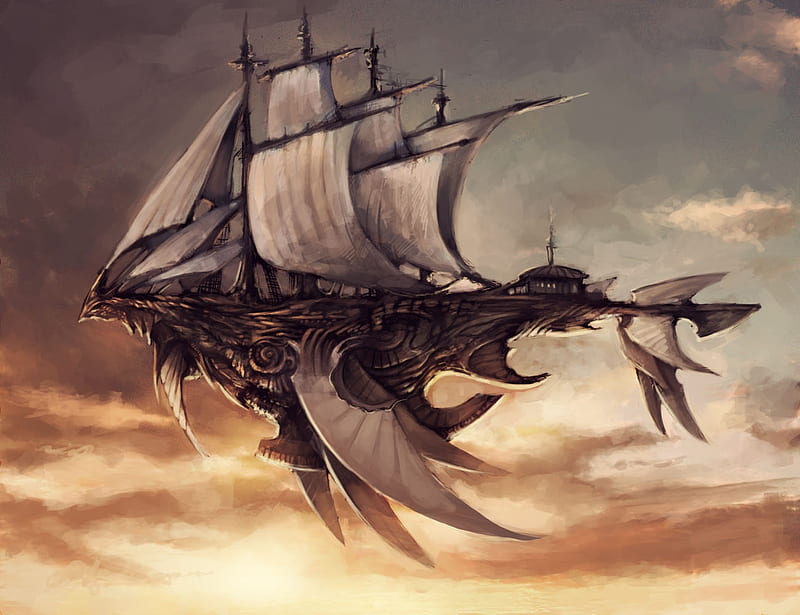The image is a detailed color illustration of a fantastical, conceptual airship soaring through the sky. The airship resembles a sea-faring sailing ship with ornately carved wooden structures, but its hull is designed to mimic an upside-down dragon's head, complete with horns, eyes, and scales. Intricately crafted, the ship boasts about eight to ten billowing, white sails unfurled from vertical dark wood masts on top, gracefully catching the wind. The main body of the ship, rendered in dark wood with lighter highlights, features wing-like appendages on the sides and at the back. These wings, along with additional fin-shaped protrusions near the front, are covered in a white canvas material. At the rear of the ship is a pointed tail, akin to a dragon's tail, adding to its mystical appearance. Nestled on the tail section, there appears to be a small house-like structure. The background sky transitions from dark and cloudy hues on the top left to a lighter, grayish tone on the top right, while the bottom of the image glows with the rich colors of a golden sunset, blending shades of yellow and orange. The airship, seemingly in motion toward the left side of the image, stands out vividly against this dramatic sky, emphasizing its fantastical and imaginative design.